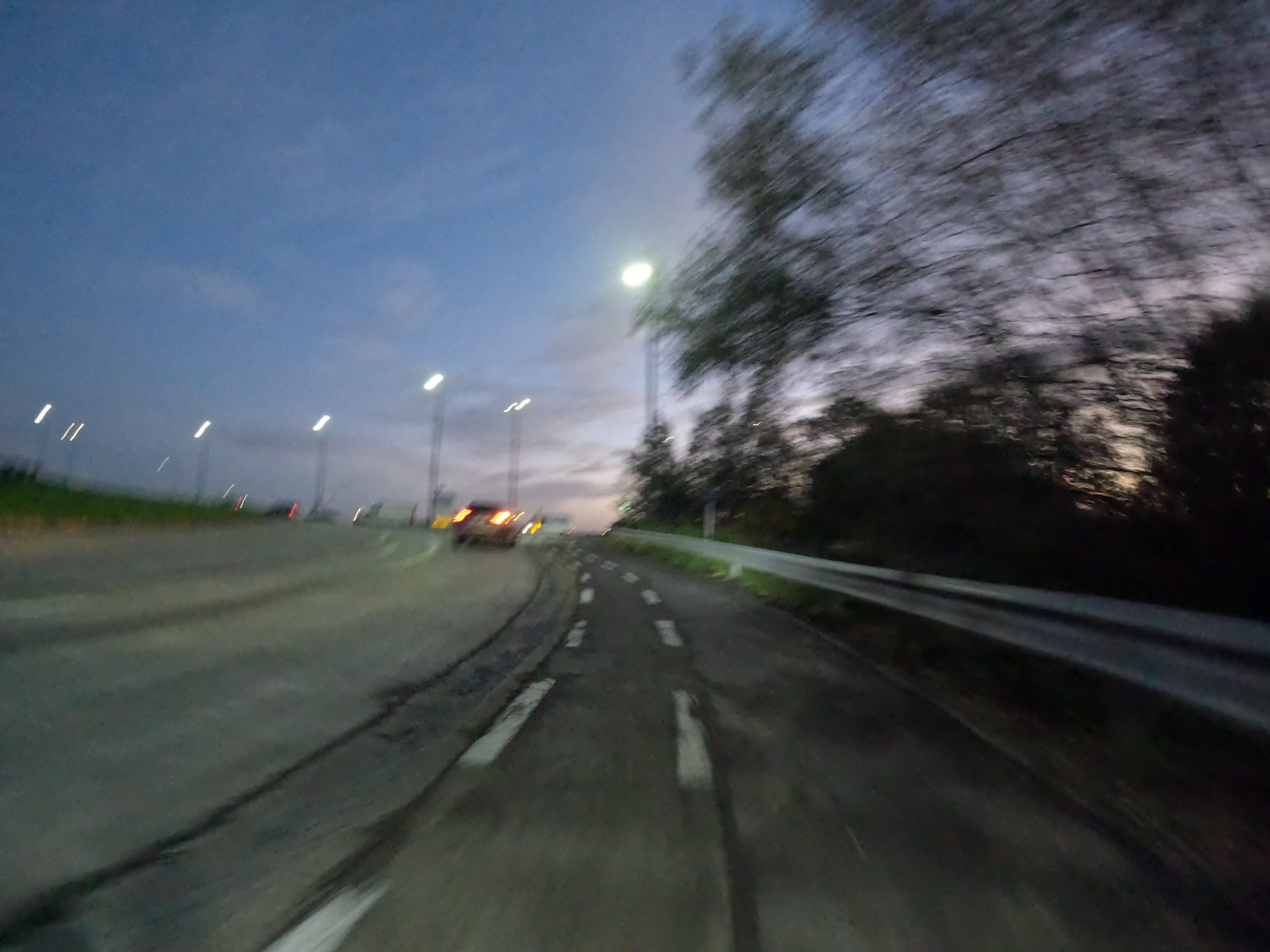This image depicts a blurry scene captured from a moving vehicle on a multi-lane highway at dusk. The gray asphalt road is marked with white lanes and flanked by a metal guardrail on the right side. Tall streetlights line the road, casting illumination on the blurred scene. In the background, a few distant cars with their taillights on can be seen, and a couple of cars are visible further down the highway. On the right side, there are trees and bushes, appearing wispy and indistinct due to the motion blur. The sky exhibits a gradient from a fading blue to golden hues near the horizon, with hints of gray clouds, indicating that the sun is setting just behind the trees. The moon has already risen, adding a subtle glow to the twilight atmosphere. The entire scene exudes the tranquility of an almost nighttime setting.